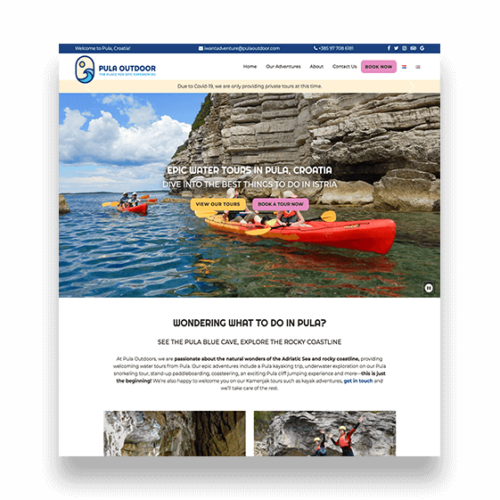The image features a header with a dark blue border containing blurry, unreadable text. Beneath this header, the text "Pula Outdoor" or "Fula Outdoor" is visible, followed by an icon depicting the Sun and an ocean wave. Directly below, a prominent purple button is displayed. 

In the central section of the image, there is a picture of people canoeing in a body of water, with a massive rock formation or mountain situated a few feet away from them. The overlay text reads, "Epic Water Tours in Pula, Croatia - Dive into the Best Thing to Do."

Additionally, there are two buttons - a yellow one and a purple one with some writing in the center. Below these buttons, more text reads, "Wondering what to do in Pula? See the Pula Blue Cave, explore the rocky coastline."

A paragraph of detailed text follows, and near the bottom of the image are two photos that have been partially cropped out.